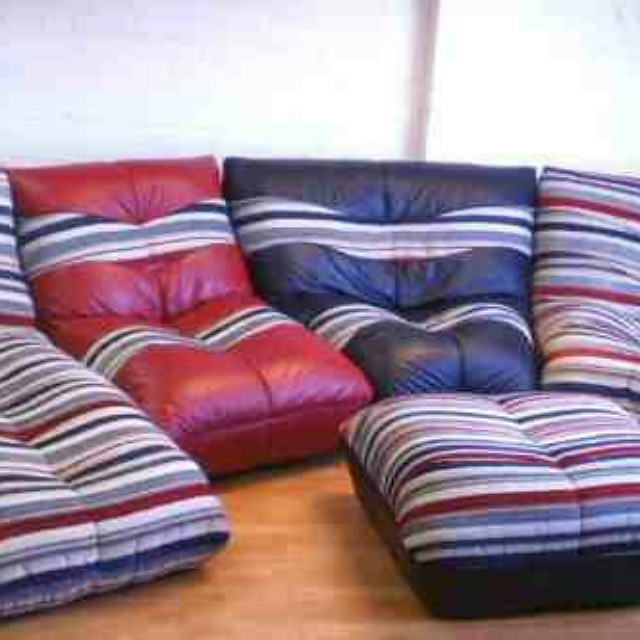The image shows a uniquely designed couch setup, composed of thick cushions with a curvy formation, all placed on a wooden floor. These cushions resemble armless couches and display a variety of colors and patterns. Two of the cushions are made from leather: one is red leather, and another is black. Intricately patterned stripes of black, white, red, and blue run horizontally across these cushions at the top and bottom. Additionally, there are similar cushions which are blue and decorated with the same stripe pattern. In front of this arrangement, there is a matching square ottoman featuring the same striped fabric and a black base. The scene is set in a room with white walls, suggesting a cozy, modern living room space.